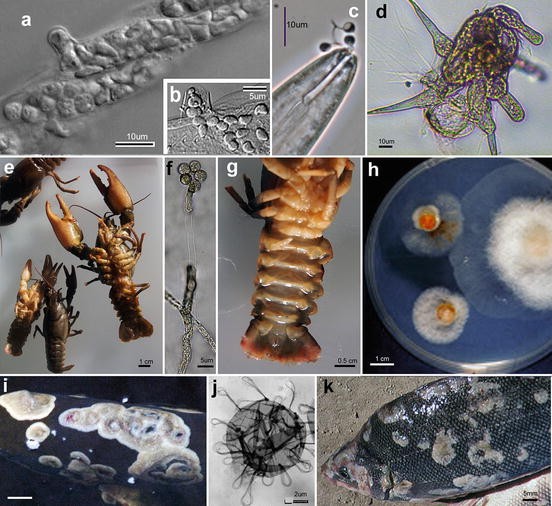This collage comprises eleven images organized into three rows and labeled from A to K. The top row features four microscopic photos of unidentified organisms, labeled A, B, C, and D, likely captured through a microscope. In the middle row, labeled E, F, G, and H, the images include identifiable marine life: a prominent lobster in box E, other crustacean-like animals in F, a lobster tail in G, and an image involving a petri dish in H. The bottom row contains three more microscopic images, labeled I, J, and K. Image K distinctly shows a fish with blue and white markings. Overall, the layout suggests the images serve an educational purpose, potentially displaying various stages of development or different magnifications of marine and microscopic life.